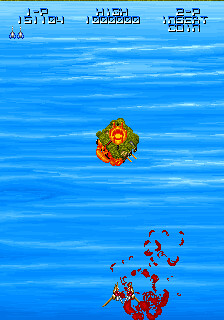The image is a screen capture from a retro video game, likely dating back to the early 80s. The majority of the background features a blue expanse that could represent either sky or sea, accented with small white highlights suggesting reflections of light. Dominating the center of the image is a square-shaped island adorned with green trees. At the heart of this island is an enigmatic red and orange circle, possibly indicative of a target or special item. In the lower right portion of the image, red streaks or marks are visible, numbering around 13 or 14 and creating a scattered, splattered appearance similar to clouds or remnants of an explosion. There may be a character or figure near the lower center of the scene, but it's indistinct. Across the top of the screen, blue and white text displays "I-P" accompanied by the score "161104." Centrally positioned is the word "HIGH" followed by "100000," denoting a high score. To the right, somewhat blurred text reads "2-P" and "insert coin." Additionally, two missile-like shapes dangle at the top left. The overall aesthetic, including the pixelated graphics and layout, clearly points to a vintage gaming style typical of early arcade games.